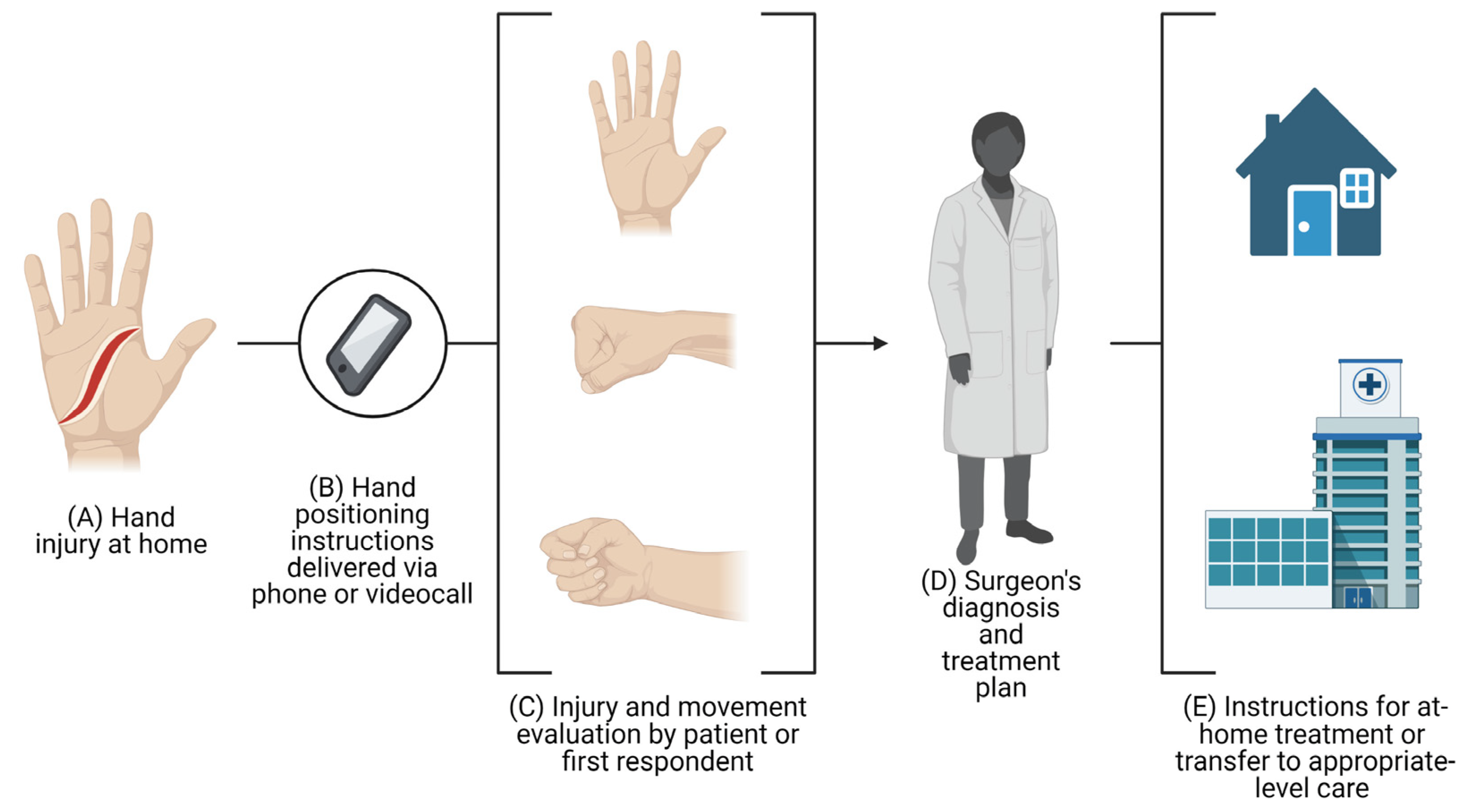The graphic artwork, labeled sequentially from A to E, provides a detailed flowchart of the steps involved in addressing a hand injury. 

(A) On the left, the first image depicts a hand with a severe cut across the palm highlighted in red, labeled "Hand Injury at Home."
(B) Next to it, an image of a black rectangular phone inside a circle represents "Hand Positioning Instructions Delivered via Phone or Video Call."
(C) The middle section shows three hand positions—a hand open, a fist in the middle, and a partially closed fist—marked as "Injury and Movement Evaluation by Patient or First Responder."
(D) Forward from that, an image of a person wearing a doctor's robe signifies "Surgeon's Diagnosis and Treatment Plan."
(E) Finally, the process culminates with an image of houses, indicating "Instructions for At-Home Treatment or Transfer to Appropriate Level Care."

Each section is connected by lines, guiding the viewer from the initial injury through to the final step in the treatment process.